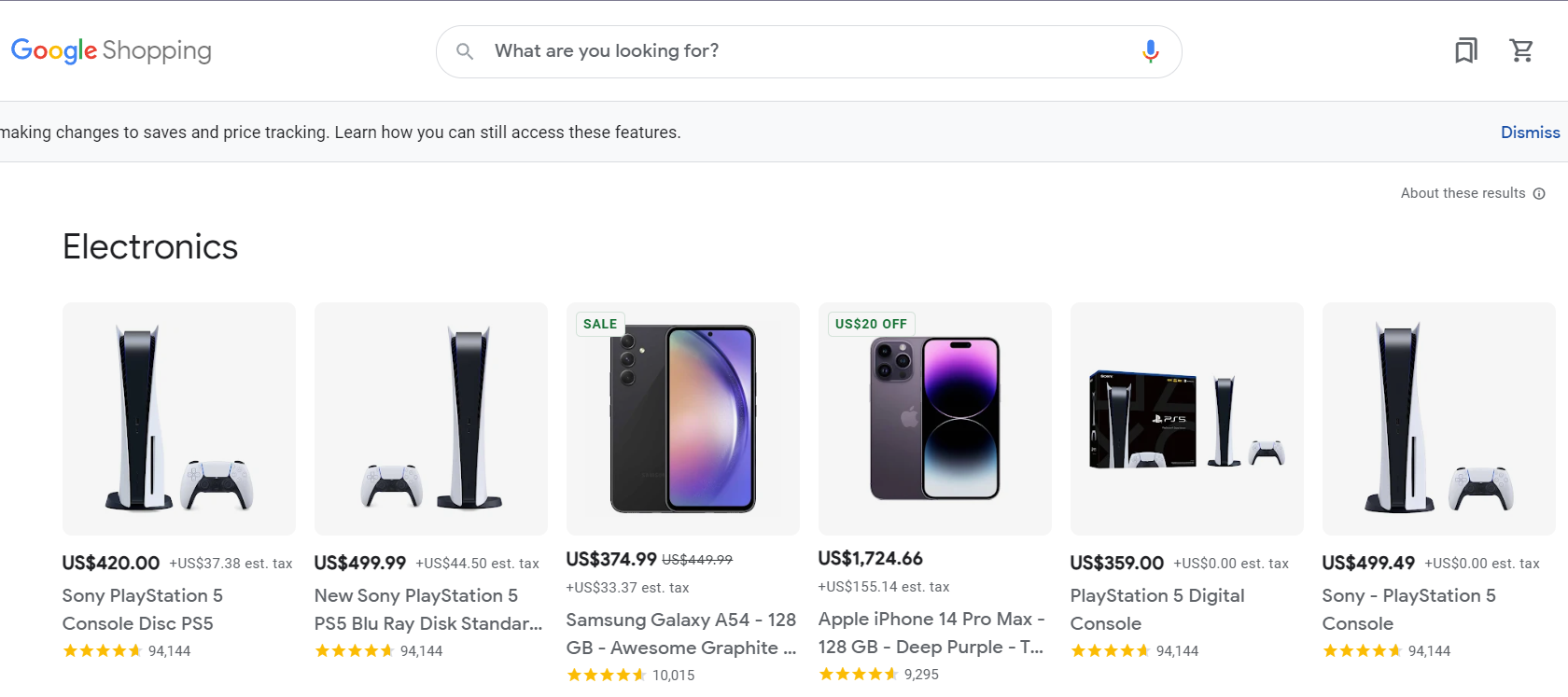This screenshot captures a section of the Google Shopping interface. At the top left corner, the multicolored "Google" logo is paired with the word "Shopping" in gray. Directly below this, a search bar features the prompt "What are you looking for?" accompanied by a magnifying glass icon and a microphone icon. To the right of the search bar, there is a bookmark icon for saving items to collections and a shopping cart icon.

Beneath the search bar, a gray notification bar informs users about "making changes to saves and price tracking" with a link to learn more about these features. To the far right of this bar, a blue "Dismiss" button is visible.

Just below the gray notification bar, an "About these results" section with an information icon allows users to click for more details. In the main content area, bold black text introduces a selection of electronics. The first highlighted item is a PlayStation 5 console disc (PS5), priced at $420.00. Next is a PlayStation 5 PS5 Blu-ray Disc Standard, listed at $499.99. The final item shown is a Samsung Galaxy A54 with 128GB of storage in "Awesome Graphite," priced at $374.99.